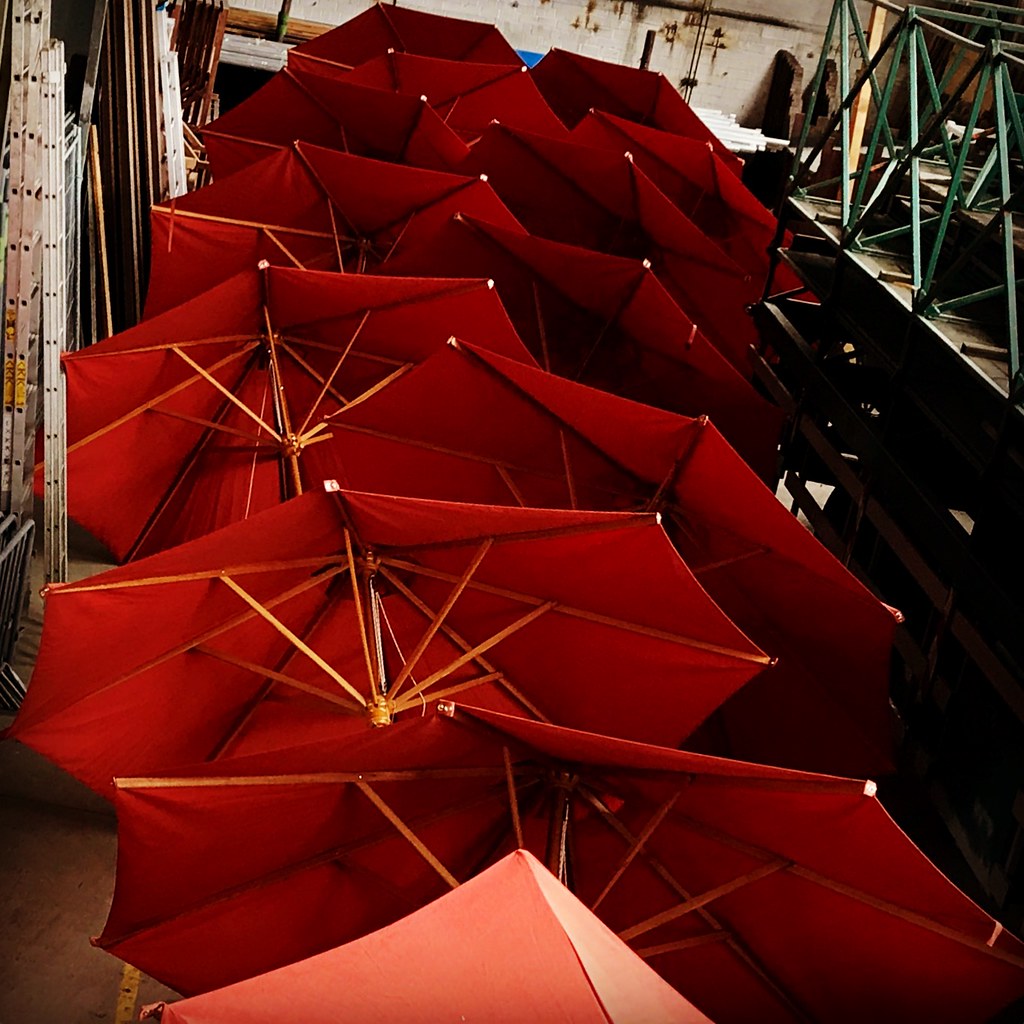The photograph captures a collection of approximately 14 large, crimson red market umbrellas with wooden poles, stacked atop one another in an almost diagonal orientation. These umbrellas are fully open and appear to be stored in a warehouse or storage room, creating a striking visual contrast with their vibrant red color against the dimmer, more muted colors of the surrounding space. Positioned vertically and overlapping each other, the umbrellas dominate the scene, with their lighter-colored wooden frames visible amidst the rich red fabric. The warehouse itself has various elements indicative of storage, including metal scaffolding in a green color on the right-hand side with an X-shaped structure, and several ladders in the top left corner. The backdrop includes white walls marred with brown stains and patches of rust, contributing to the overall industrial and utilitarian atmosphere of the setting.